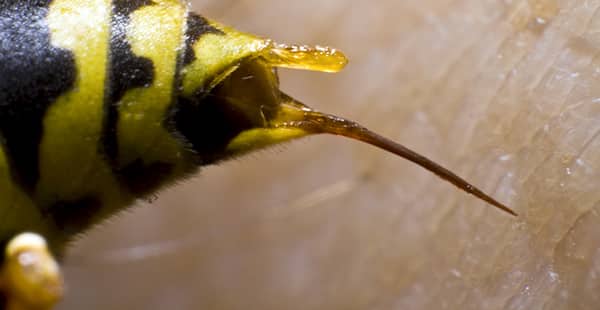The image is an extreme close-up, horizontal color photograph featuring the back end of a bee, possibly a wasp or hornet, poised to sting human skin. The insect, characterized by its shiny black and yellow striped abdomen, dominates the top left of the image. Its menacing stinger, elongated and sharp, protrudes purposefully from the hind end, almost touching the pinkish-beige skin that forms the backdrop. The skin, detailed with tiny hairs, hints at the stinger's imminent piercing action. This visually striking photograph captures the tense moment just before the insect's stinger makes contact with the human skin.